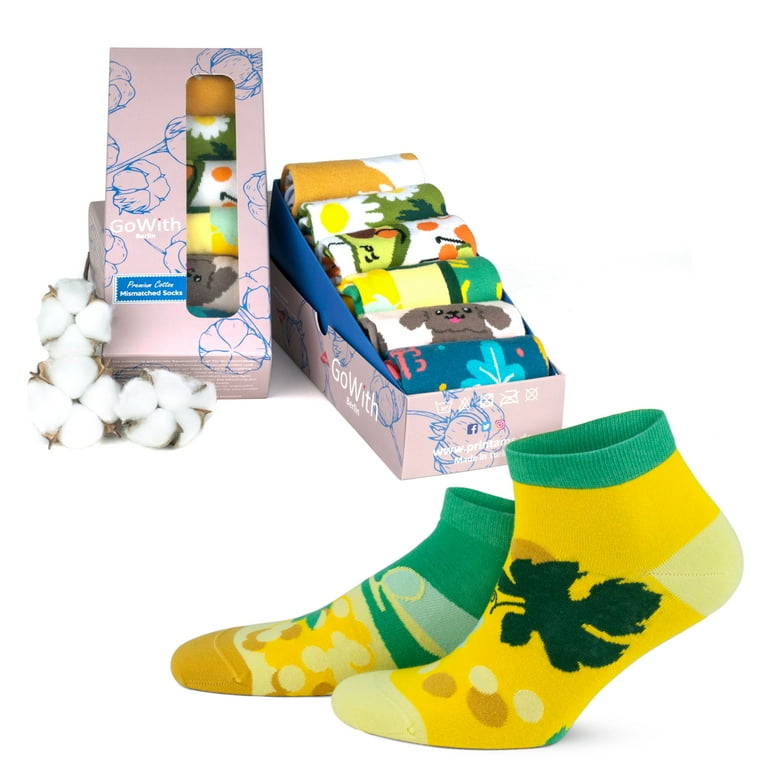This professionally photographed product image showcases a vibrant collection of socks set against a clean white background, likely taken in a studio. In the foreground, a pair of mismatched quarter-length socks display a harmonious blend of teal, yellow, goldenrod, and white, featuring brown and tan circular patterns and a prominent gray leaf design. 

Behind these, two pink boxes labeled "Go With Socks" contain six neatly rolled socks, each exhibiting playful and colorful designs like smiling dogs, avocados with arms, and white daisies against green backgrounds. To the left of these boxes, sprigs of cotton are delicately placed, hinting at the socks' cotton composition. The image also includes subtle social media icons on the box, reinforcing its promotional purpose.